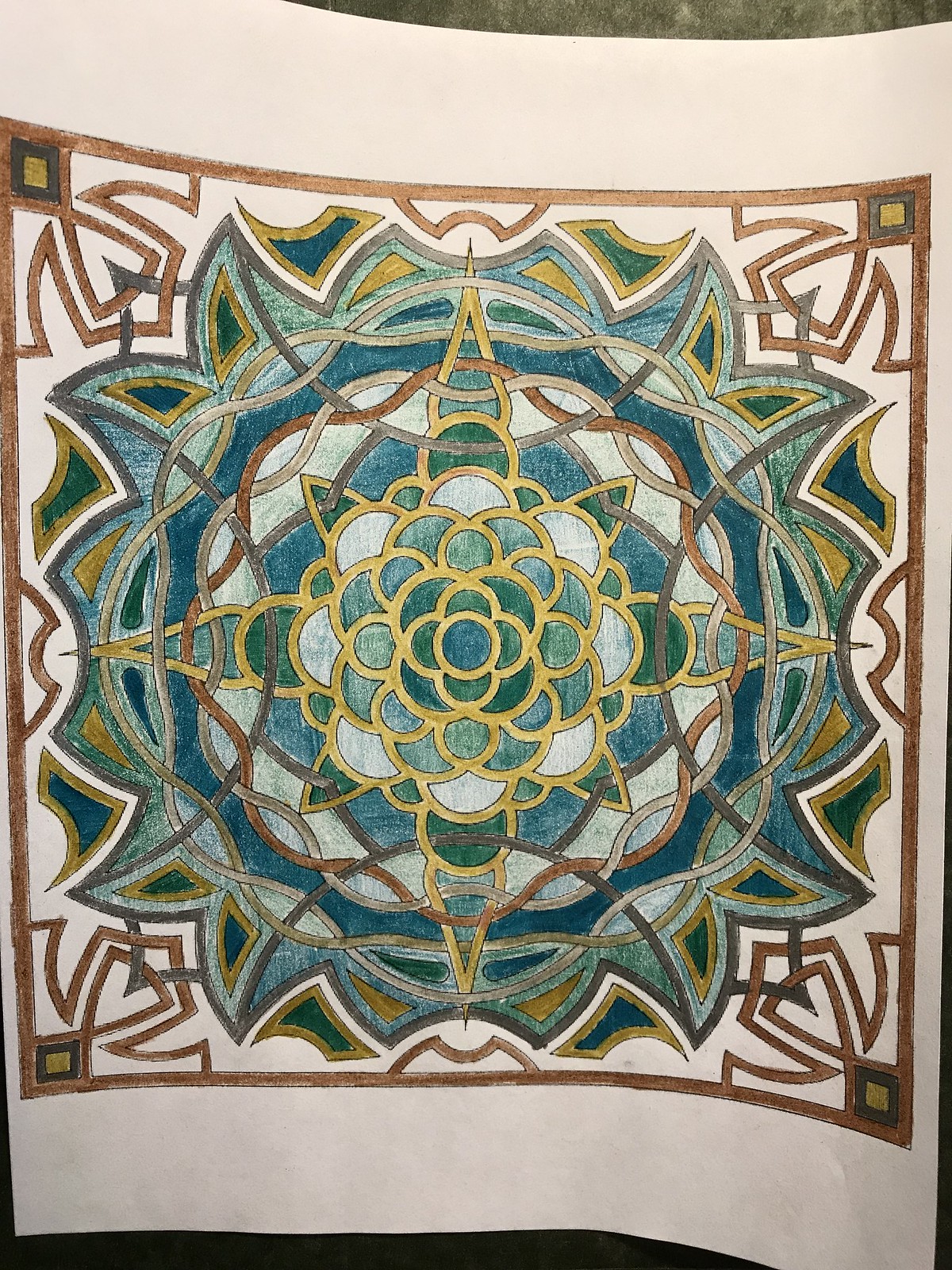The image captures an intricately detailed piece of artwork on a slightly curved, light gray or dusty rose-colored sheet of paper. Resting on dark surfaces, the artwork exhibits a mandala-like design, typical of adult coloring books meant for relaxation. The outer boundary features a brown square with smaller squares at each corner, filled with gold and brown square patterns. From the squares, brown leaf shapes extend outward. Moving inward, green fragments bordered with gold dominate the middle sections. At the center, a mini-star shape edged in gray encases a blue filling adorned with additional gold patterns. The focal point concludes with a four-cornered star shape enveloped by cloudy, gold-bordered designs. Various shades of blue, greenish-blue, turquoise, bronze, and gray paint the intricate floral and geometric motifs, likely hand-colored with pencils or markers. The complex, rosette and mosaic-like patterns evoke a mix of traditional and Native American-inspired elements, intertwining repetition and stylized curls in a meticulous and calming composition.